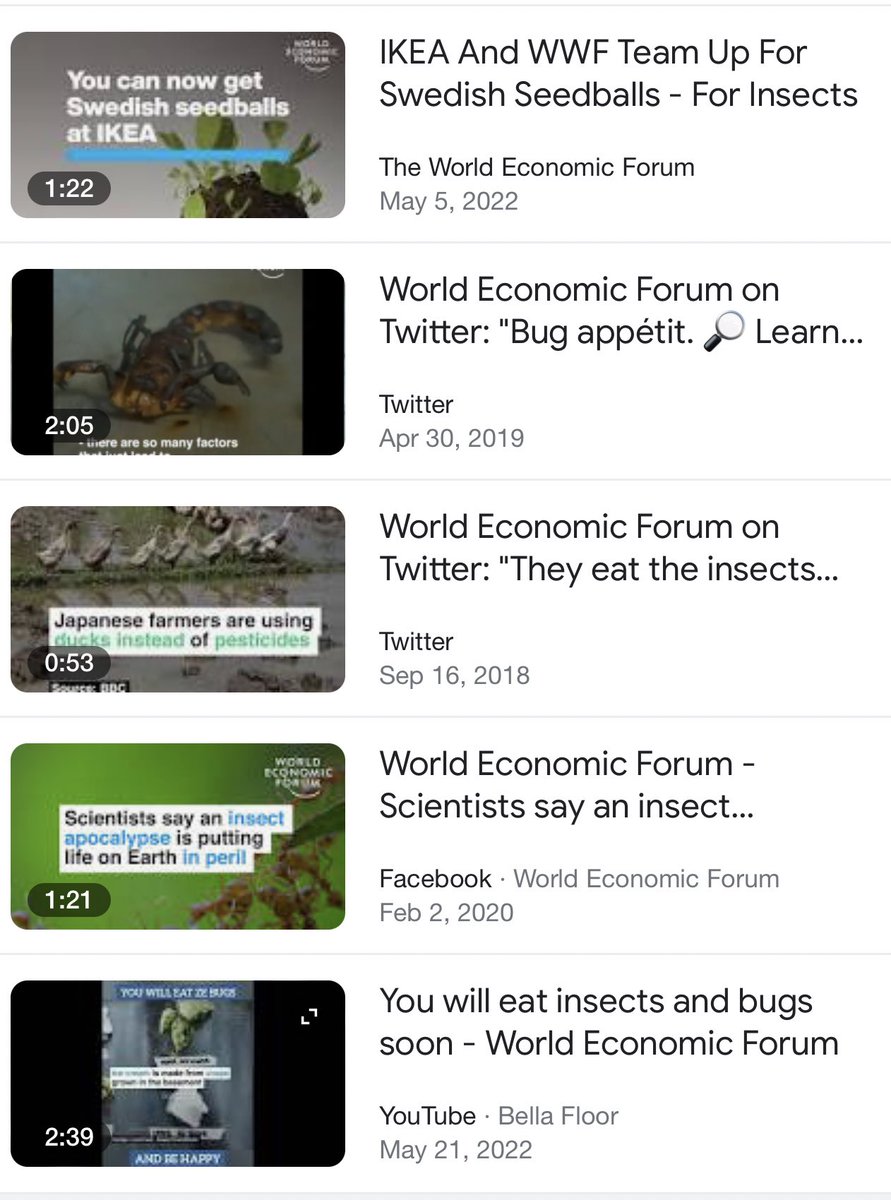The image appears to be a desktop or tablet screenshot displaying a selection of videos. Due to the partial view, the precise nature of the application or web browser and the operating system cannot be identified. The content predominantly features videos related to the theme of insects, many of them courtesy of the World Economic Forum. 

**Detailed Caption:**

The screenshot captures a video playlist interface, likely from a desktop or tablet screen. The first video, entitled "You can now get Swedish seed balls at IKEA," is 1 minute and 22 seconds long and presents a plant against a gray backdrop. The associated text highlights a collaboration between IKEA and the World Wildlife Federation (WWF) to promote Swedish seed balls for insects, with the World Economic Forum mentioned as well (May 5th, 2022).

The second video, lasting 2 minutes and 5 seconds, features an image of a scorpion. Part of the caption reads, "There are so many factors…" with the full context obscured. The video, sourced from the World Economic Forum's Twitter, discusses entomophagy under the title "Bug appetite with a magnifying glass," dated April 30th, 2019.

The third video shows a pond with several ducks in a 53-second clip. Captioned "Japanese farmers are using ducks instead of pesticides," the video explains that ducks consume insects, aiding pest control. This video is marked as a World Economic Forum post from Twitter, dated September 16th, 2018.

The fourth video is 1 minute and 21 seconds long and displays ants on a leaf. It brings attention to the potential "insect apocalypse" threatening Earth's ecosystem, with the accompanying text pointing to scientific concerns shared by the World Economic Forum. The video is tagged as a Facebook entry, sponsored by the World Economic Forum from February 2nd, 2020.

The final visible video, with a duration of 2 minutes and 39 seconds, appears to be a cell phone recording. It references the promotion of insect consumption, with phrases like "You will eat ze bug and be happy" and "You will eat insects and bugs soon." This content is noted to be from a YouTube video via Bellaflore, dated May 21st, 2022.

Overall, the screenshot collectively showcases a series of videos discussing various aspects of entomophagy and the ecological roles of insects, emphasizing educational and promotional content from the World Economic Forum.